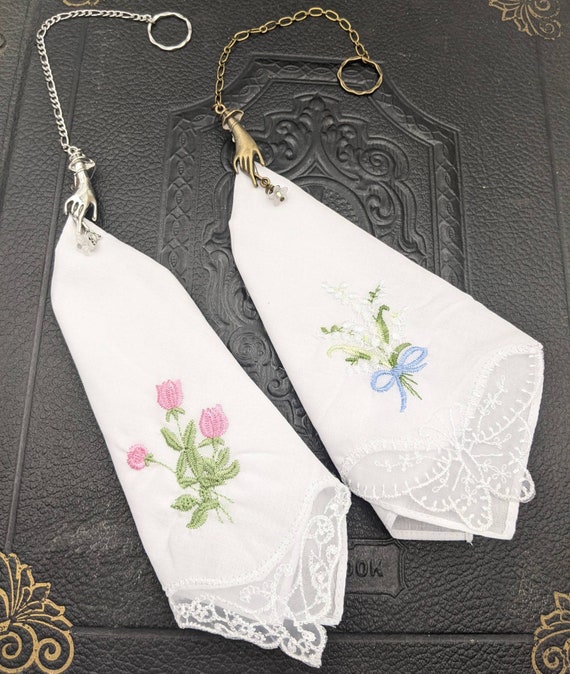The image displays two intricately embroidered lady's handkerchiefs, known as Kurchis, each adorned with delicate floral designs. One handkerchief features pink roses accompanied by green leaves, while the other showcases white flowers with green leaves and a small blue bow. Both are expertly folded and held in place by elegant clips—one shaped like an animal in silver, and the other like a woman's hand in gold. These clips also incorporate tiny flower motifs that match the color of the chains attached to them. The handkerchiefs rest on a richly etched leather book, which bears gold designs in its corners and partial, unreadable text ending with either "O-W" or "O-K." The book's sophisticated appearance complements the refined presentation of the handkerchiefs.